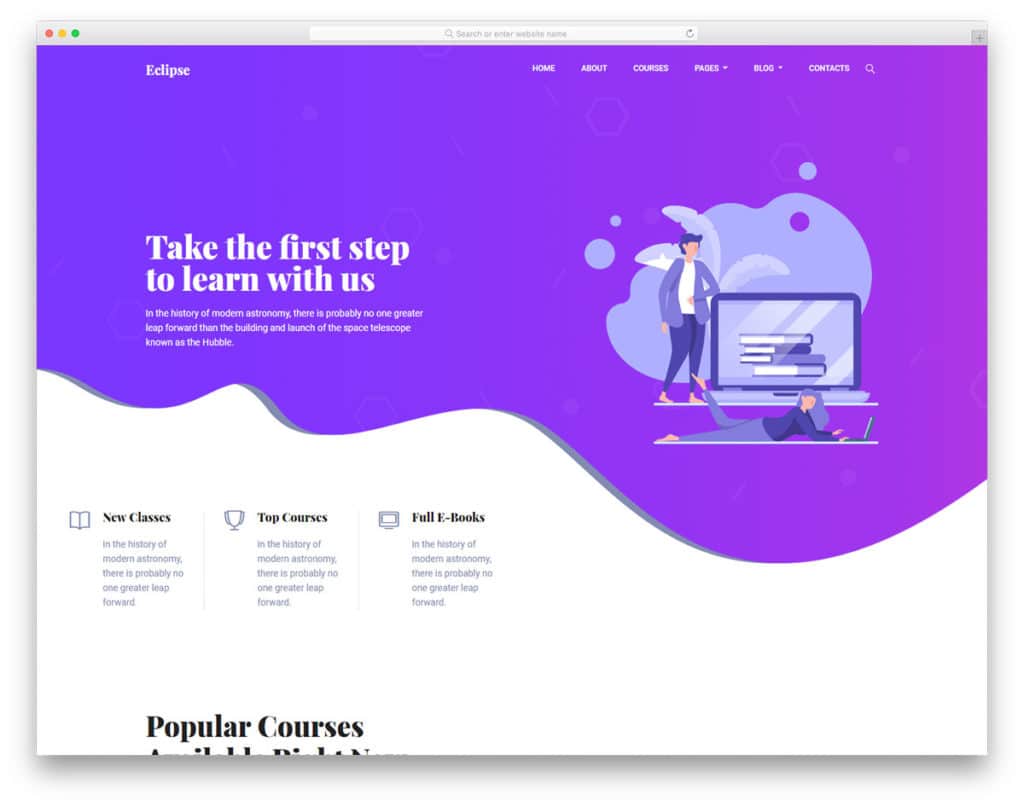The image appears to be a screenshot taken on a Macbook or an Apple computer, identifiable by the distinct red, yellow, and green buttons in the top left corner. The screen displays a webpage from Eclipse, an educational platform. The website's navigation bar features tabs labeled Home, Courses, Pages, Blog, and Contacts. A prominent section on the page encourages users to "Take the first step to learn with us."

Multiple sections on the webpage emphasize the importance of modern astronomy, particularly highlighting the monumental achievement of launching the Hubble Space Telescope. Repeated phrases such as "In the history of modern astronomy, there's probably no greater leap forward..." underscore this point.

The page also includes dedicated sections for New Classes, Top Courses, and Full E-books, each reiterating the aforementioned importance of modern astronomy. Towards the bottom of the screen, partially visible text hints at a section for Popular Courses. Additionally, the webpage features graphics depicting two individuals next to laptops, reinforcing the educational and online learning theme of the site.